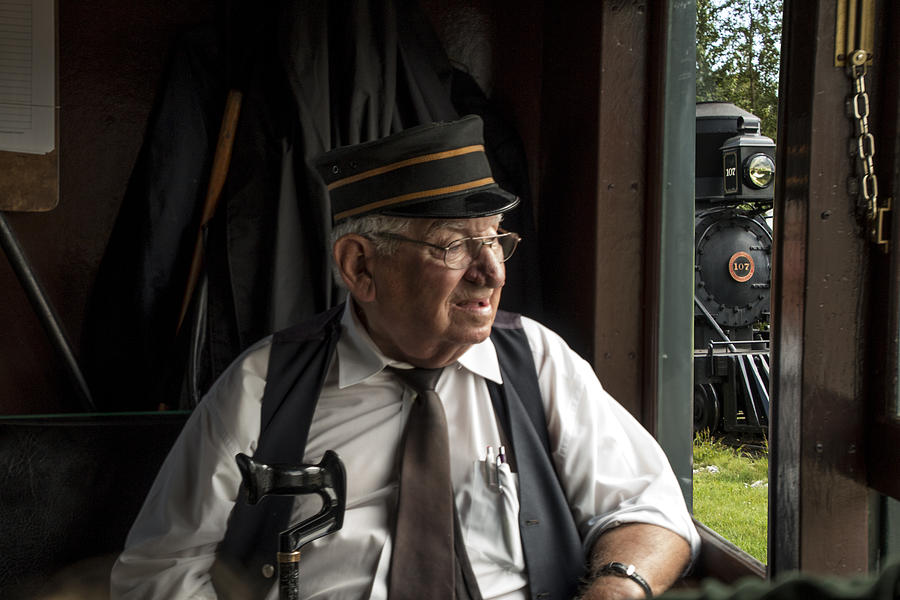The image features an elderly man, prominently positioned in the center, sitting in what appears to be a train car. He is wearing a traditional conductor's outfit, which includes a black conductor cap with yellow-orange stripes and a black vest over a white button-down shirt accompanied by a brown tie. The man has glasses, white hair, and his mouth is slightly open as he gazes out of the window, giving an impression of contemplation or reflection. A black cane is held in his hands and he has pens sticking out of his shirt pocket, along with a watch on his wrist. Behind him, through the window, the front engine of an old-fashioned steam train can be seen. The train is black with a distinctive circular number plate in orange displaying the number 107. In the background of the interior, there appears to be a hanging area possibly for coats or a schedule peeking out from the corner, adding to the nostalgic and historical ambiance of the setting.